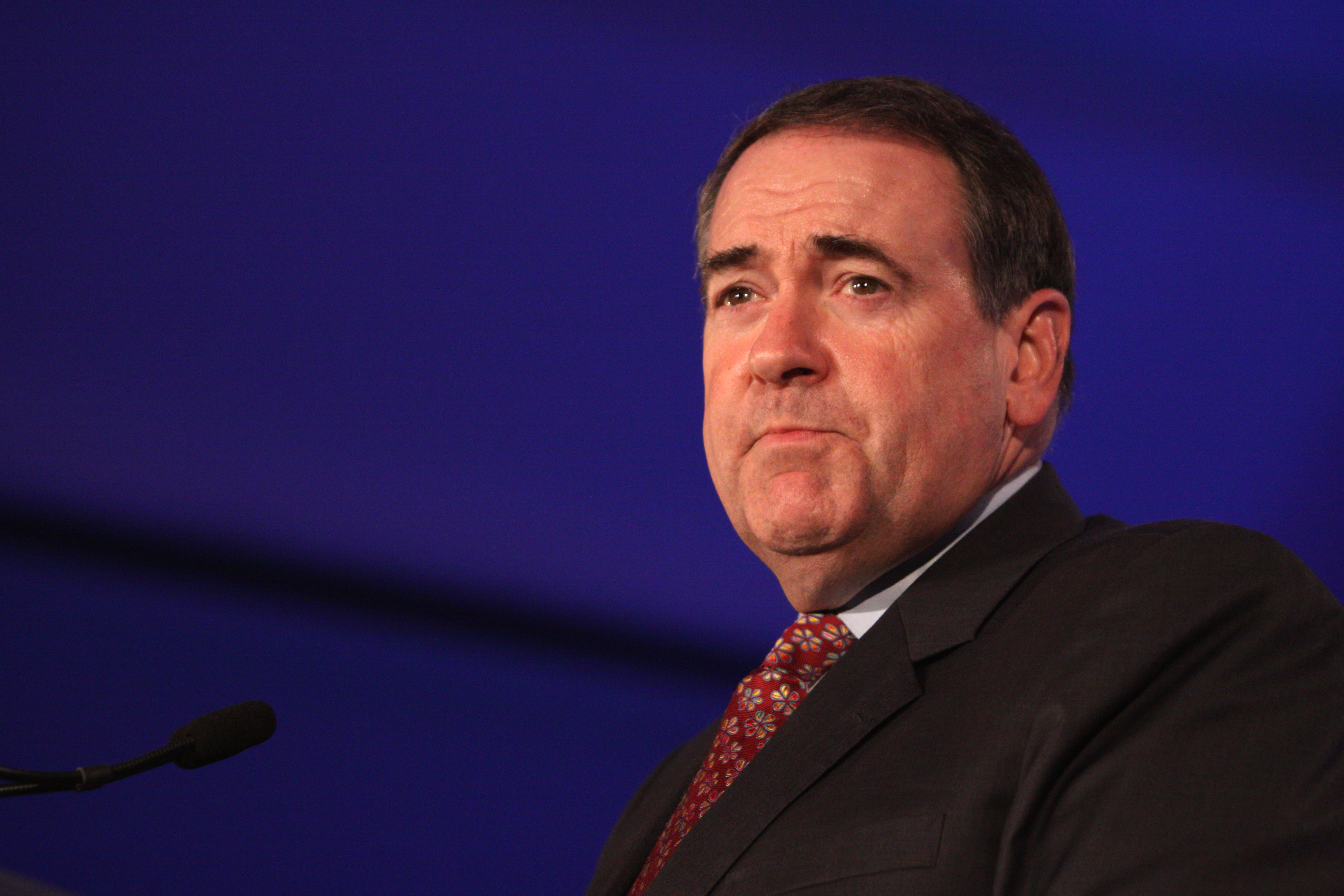This photograph captures a middle-aged Caucasian man, likely in his late 50s, with dark brown hair and brown eyes, standing against a partially illuminated blue wall with a black stripe. He appears heavyset and is dressed in a black suit jacket paired with a distinctive red tie adorned with blue, red, and yellow floral patterns. The man, who resembles Mike Huckabee, is positioned behind a black microphone located at the bottom left corner of the image, suggesting he is giving a speech. He is not looking directly at the camera, but rather staring off into the distance, adding an air of contemplation. The setting and his formal attire imply he might be a notable politician or a business leader.